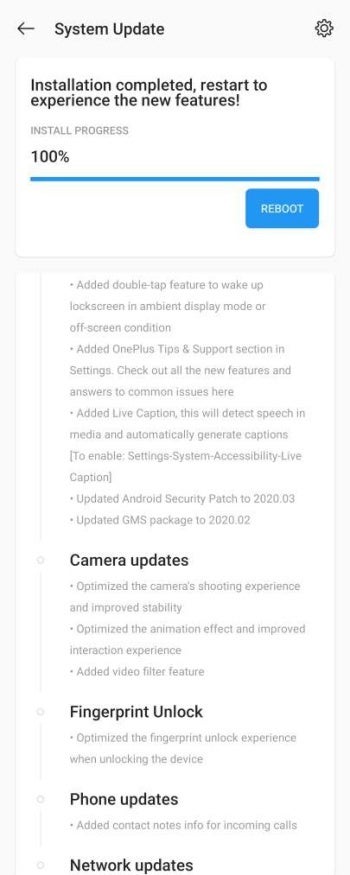The image features a predominantly white background with black text and several interface elements, giving the impression of a software update notice or settings update screen.

At the top left corner, there is a black button featuring the label "System Update" to its right. On the opposite corner, the top right, sits a black gear icon, indicating access to settings.

Just below this top section, the main body of the message begins with the text "Installation completed. Start to experience the new features." This is followed by "Install progress: 100%". A blue progress bar spans across the screen, completely filled, signifying the completion of the installation process. To the bottom right of this progress bar, a blue button labeled "Reboot" is prominently displayed.

The lower portion of the image is densely populated with descriptive text outlining the new features and updates included. This section reads as follows:

- **Edit double tap feature**: Tap twice to wake up the lock screen in ambient display mode or off-screen condition.
- **Edit OnePlus tip and support section in settings**: A new section to explore all the new features and find answers to common issues.
- **Edit live caption**: Detects speech in media and automatically generates captions. Enable this via Settings > System > Accessibility > Live Caption.
- **Security Updates**: Updated Android security patch to March 2020.
- **GMS Package**: Updated to February 2020.
- **Camera update**: Optimized the camera's shooting experience and improved stability. Enhanced animation effects and interaction experience.
- **Edit video filter feature**: Details not provided.
- **Fingerprint unlock**: Optimized the experience of unlocking the device using the fingerprint sensor.
- **Phone update**: Add contact note information for incoming calls.
- **Network update**: Details not provided.

The text ends rather abruptly with "Network update," indicating that further details or descriptions may have been omitted or are not applicable.

Overall, this image appears to be a detailed update log or notification for a software update, likely from a OnePlus device, introducing various system enhancements and new functionalities.